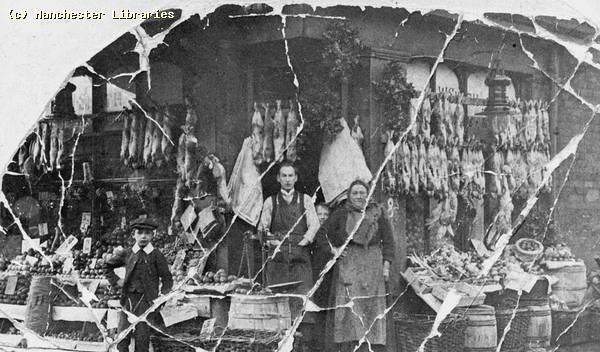This old black-and-white photograph, likely dating from the late 1800s to the early 1900s, is sourced from the Manchester Libraries. The aged image, possibly a glass plate photograph, shows signs of wear with visible lines and cracks. The scene captures a small shop, perhaps an early grocery store, with various goods displayed outside in baskets, barrels, and crates. Hanging from the eaves are what appear to be meats, possibly chickens or rabbits, and an assortment of fruits and vegetables are laid out on tables in front of the store.

In the photograph, there are four figures facing the camera with serious expressions. On the far left stands a young boy, dressed in a dark suit with a white collar and a dark cap, his right hand placed confidently on his hip as he leans against a crate. Central to the image is a shopkeeper, identifiable by his apron, and next to him a woman also wearing an apron, indicative of their roles within the store. Between them, a less visible child peeks out shyly. The detailed attire of the individuals and the assortment of goods eloquently capture a snapshot of everyday life from a bygone era.